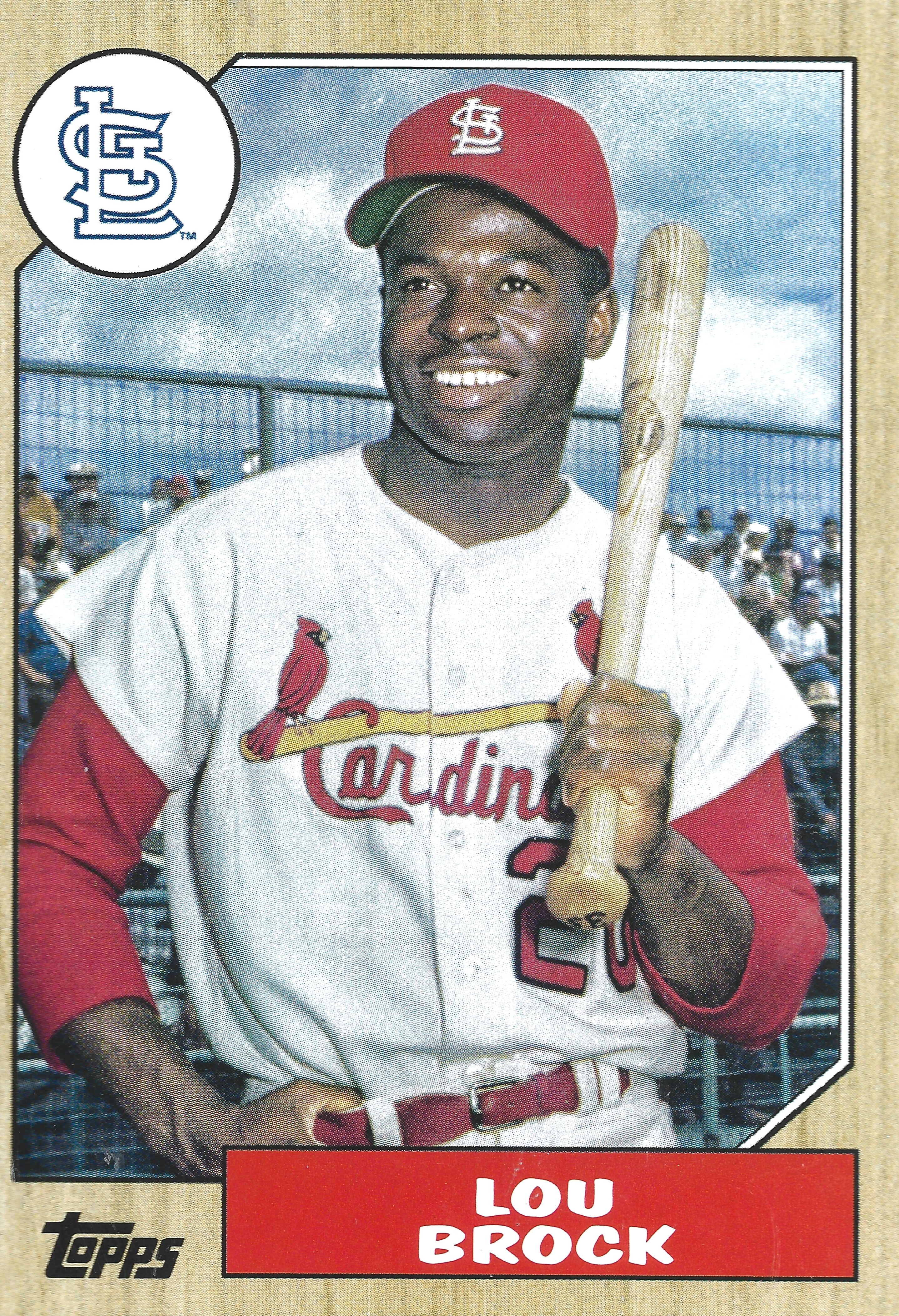The image depicts an old-timey Topps baseball card featuring Lou Brock of the St. Louis Cardinals. The card has a distinctive brown border with a grainy texture resembling a baseball bat, thicker at the top and bottom. At the upper left corner, encased in a white circle with a blue trim, is the St. Louis Cardinals logo showcasing the intertwined 'S' and 'L'. Lou Brock, an African American man, is at the center of the image, posed from head to just below the waist. Dressed in a white Cardinals uniform with red lettering and two red Cardinals perched on a yellow branch, he holds a bat upright on his left shoulder with his left hand, his elbow slightly bent. He sports a red Cardinals cap featuring the 'SL' in white text. The bottom right corner of the card displays his name, "Lou Brock," in white font set against a red rectangle, with "TOPPS" denoted in black text at the bottom left. The background includes a visible crowd and a clear sky, accentuating the nostalgic feel of the card.